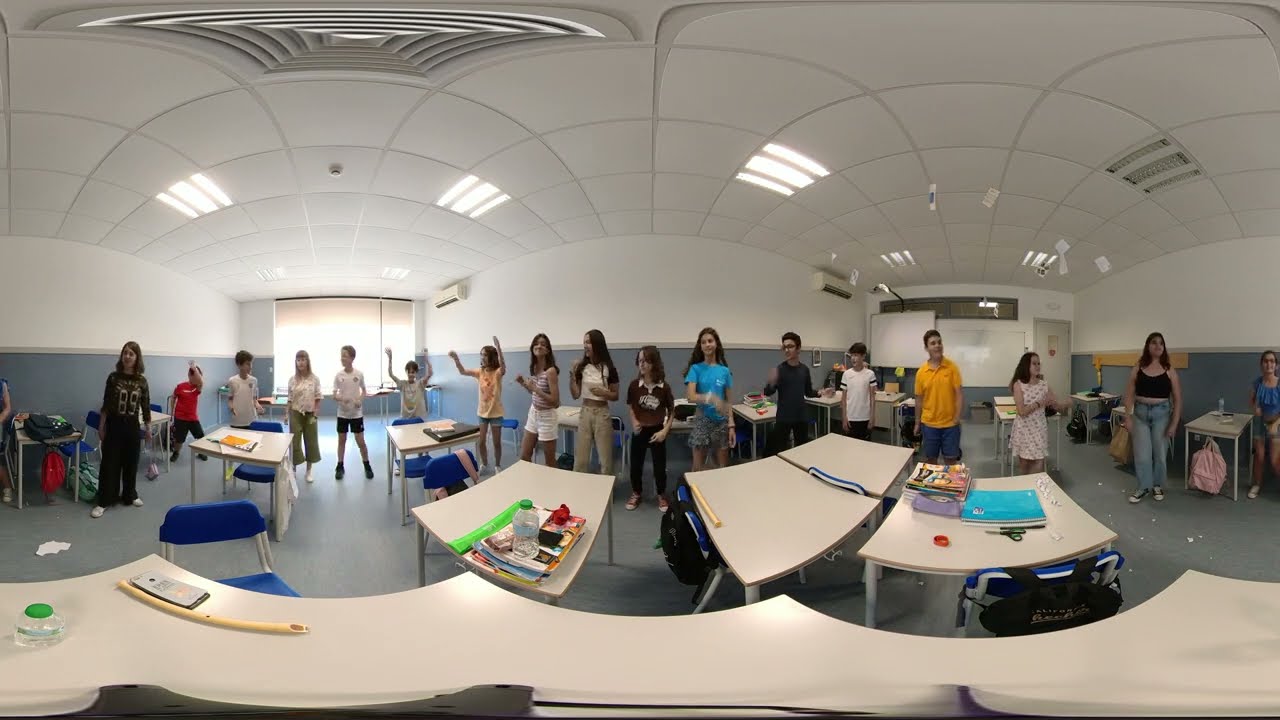The image depicts a classroom with white walls, gray borders, and a gray floor. The ceiling, adorned with tile designs, features fluorescent lighting and visible vents, indicating a 360-degree camera effect that warps the ceiling slightly. At the back of the classroom, a large window provides natural light. The children, appearing to be around 10 years old, are all standing in line facing the camera, dressed in shorts or pants and sleeveless shirts or t-shirts. Surrounding them are individual desks and larger tables, all accompanied by blue chairs. Various backpacks are scattered on the floor and atop desks, along with books and other school supplies. The overall scene suggests a pause in classroom activity, possibly for a presentation or photo opportunity.